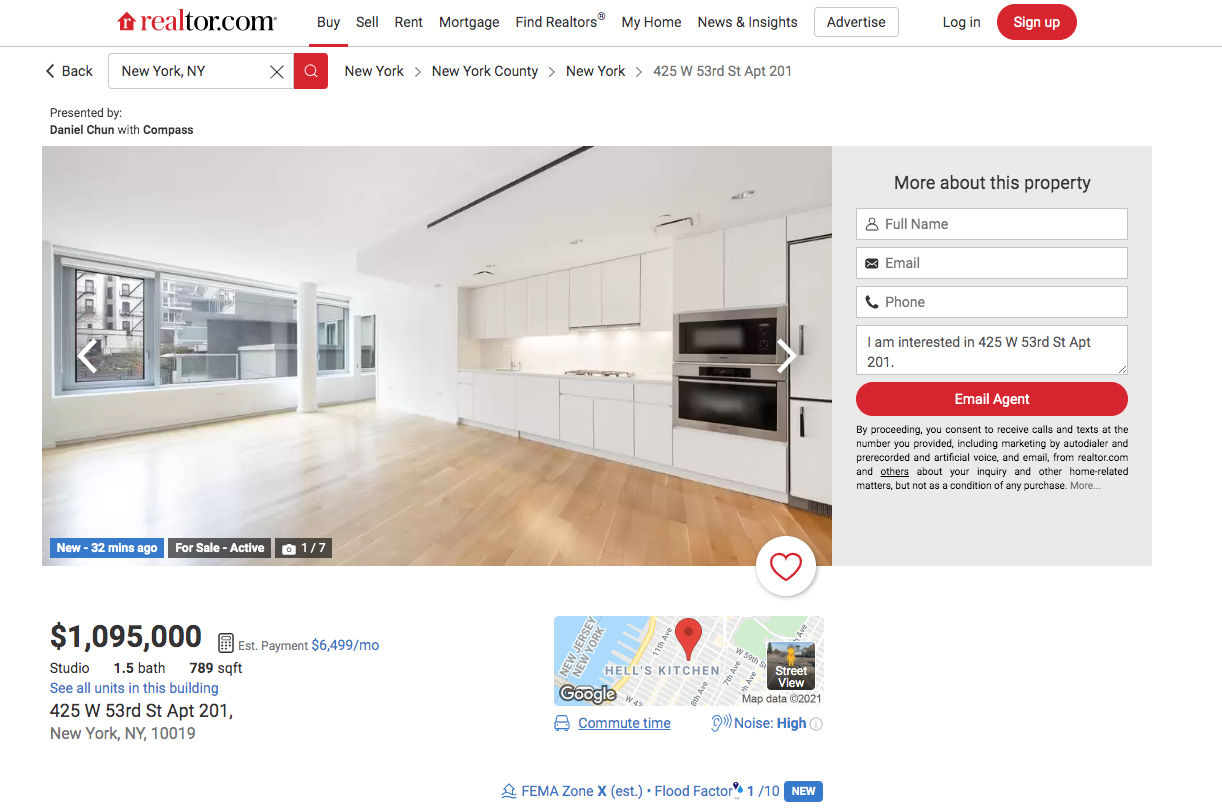The webpage depicted is from Realtor.com. At the top of the page, there is a navigation menu featuring various options: Buy, Sell, Rent, Mortgage, Find Realtors, My Home, News and Insights, and Advertise. Additionally, users can see a Login option and a prominent red Sign Up button. The location specified is New York, New York, highlighted in a red search box, with listings for New York County and the address 425 West 53rd Street, Apartment 201.

This particular listing is presented by Daniel Chun with Compass. The property is priced at $1,950,000, offering a studio layout with one and a half baths, over 789 square feet. There is a button labeled "See All Units in this Building" for more options. The estimated monthly payment for this property is $6,499.

A map on the page includes icons from Google and Street View, displaying additional data like commute time, noise level rated as high, and a flood factor of 1 out of 10. The majority of the webpage has a clean, white background.

An image of the apartment showcases its interior, featuring hardwood flooring, white cabinets, and a large window providing ample natural light.